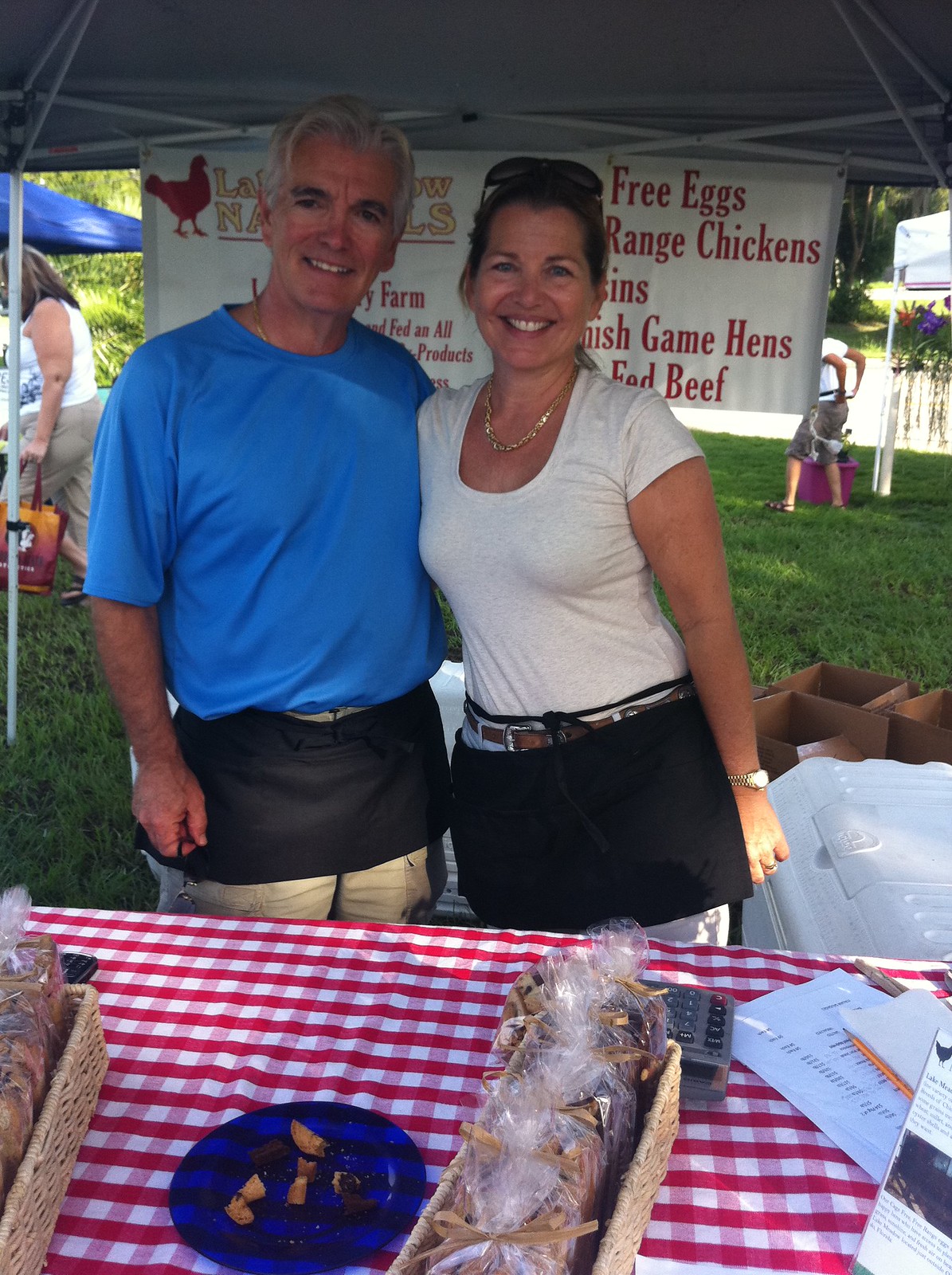The photograph captures a cheerful man and woman standing together under a large tent on a sunny day, likely at a food market or fair. Both are clad in black aprons, presumably indicating they are either selling or serving food. The man, with grayish white hair and a bright blue shirt, stands to the left, while the younger woman, who has dark brown or black hair and sunglasses perched on her head, sports a white scoop-neck, short-sleeve shirt, and stands to the right. They smile warmly at the camera, positioned in front of a table adorned with a red and white checkerboard picnic tablecloth. On the table, there are a blue plate with food samples, wicker baskets containing packaged food items possibly including bread, a calculator, a pencil, and some papers. A sign behind them advertises “Cage-free eggs, Range chickens, Cornish game hens, and Grass-fed beef,” partially obscured but clear, with a red chicken logo on the left. People can be seen walking in the grassy background, contributing to the lively outdoor atmosphere.